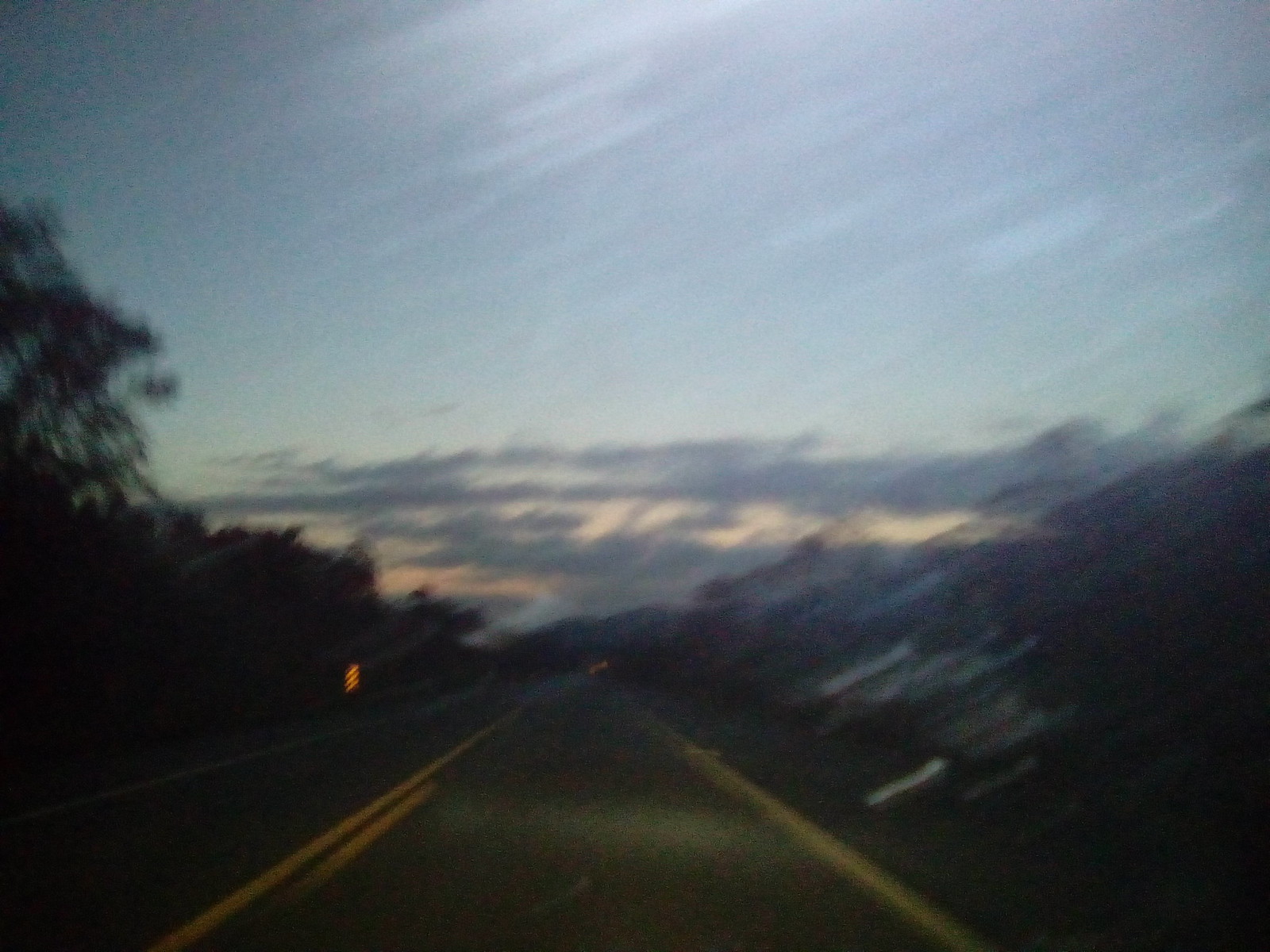A slightly blurry photograph captures the perspective of someone driving down a rural road. The image shows a captivating scene where the horizon exhibits a beautiful blend of yellow and peach hues, indicating either a sunset or sunrise. Dark clouds loom in the distance, contrasting with the colorful sky. Through the windshield, streaks of blue or possibly the encroaching night sky add depth to the view. 

The road itself is marked with multiple double yellow lines, suggesting a well-traveled pathway that stretches endlessly into the countryside. Flanking the road, diverse shrubbery and trees create a natural, untamed border. Among these, a red and white flag marker stands out, subtly illuminated on the left side of the road, adding a touch of human presence to the otherwise serene landscape.